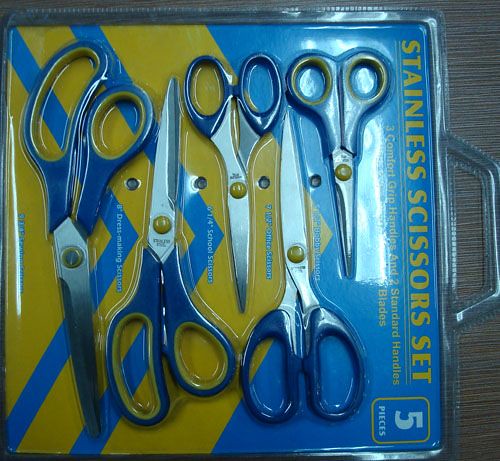This is an image of a set of stainless steel scissors, each with distinct blue and yellow handles, neatly arranged within a clear plastic clamshell packaging that features a convenient handle on the right. The packaging predominantly showcases a turquoise blue background at the top, which prominently displays the label "Stainless Scissors Set" in yellow, accompanied by smaller yellow text indicating "comfort grip handles and two standard handles." The lower section of the packaging features a yellow triangle with two blue chevrons, enhancing the package's colorful appeal. In the center of this yellow triangle, bold white text announces "five pieces." The set includes three pairs of scissors with comfort grip handles, well-padded in yellow, and two pairs with standard blue handles. Each of the scissors is fastened by a conspicuous yellow rivet. The assortment varies in size, ranging from a large dressmaking shears to a tiny pair ideal for precise tasks like hair-trimming.